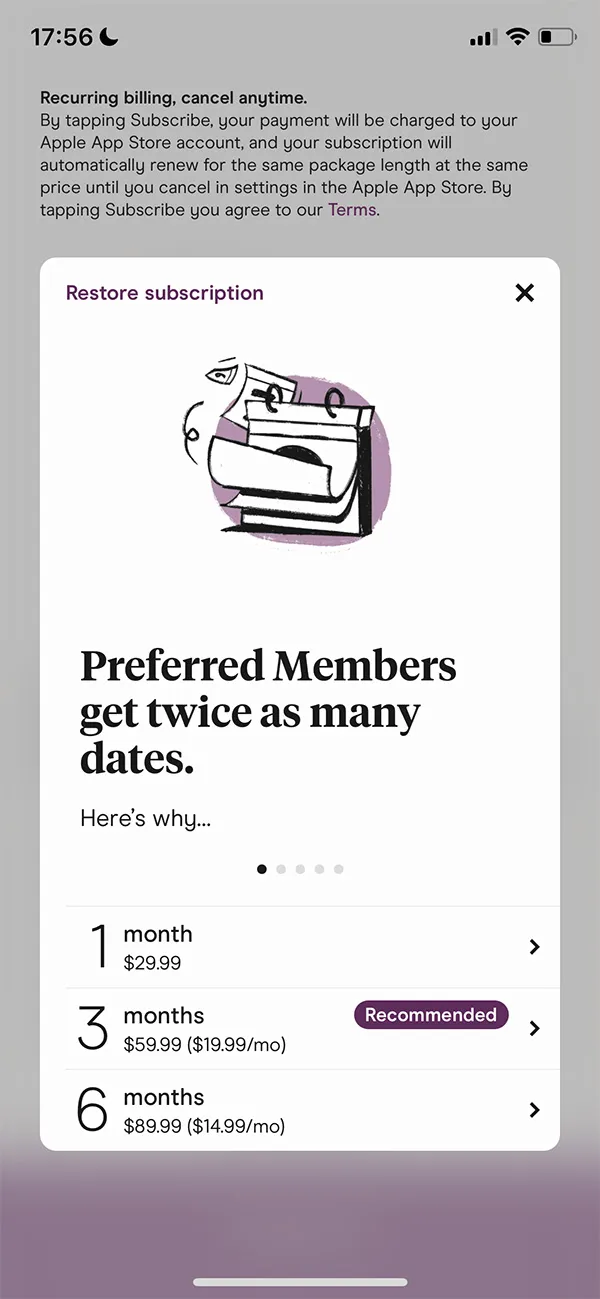The image showcases a detailed mobile screenshot. 

### Upper Section:
- **Top Bar:**
  - **Left:** Time displayed as 17:56 in black text, accompanied by a black crescent moon icon.
  - **Right:** Icons for Wi-Fi and battery status.

### Main Background:
- **Title Area:**
  - **Text:** "Recurring Bill, Cancel Anytime" in bold black font.
  - **Subtext:** Notice in less bold black letters stating, "By tapping Subscribe, your payment will be charged to your Apple App Store account, and your subscription will automatically renew for the same package link at the same price until you cancel in settings from the Apple App Store. By tapping Subscribe, you agree to our terms," with "terms" highlighted in purple, indicating a hyperlink.

### Popover Box:
- **Top Bar:**
  - **Left:** "Restore Subscription" in dark purple font.
  - **Right:** A black exit 'X' icon.
- **Middle Section:**
  - **Icon:** Light purple circle with turning white calendar pages inside.
  - **Heading:** "Preferred Members Get Twice As Many Dates" in bold black font.
  - **Subheading:** "Here's Why" in smaller, less bold black font.
  - **Navigation Dots:** Five circles in total; the first is black, the rest are gray, indicating page progression.
- **Separator:** Thin gray borderline.

### Subscription Options:
- **Option 1:**
  - **Duration:** "1 Month" with "29.99" cost in black text.
  - **Arrow/Caret:** Black caret pointing to the right.
  - **Separator:** Thin light gray line.
- **Option 2:**
  - **Duration:** "3 Month" with "59.99" cost in black text and "$19.99/Month" in parentheses.
  - **Recommended Label:** Placed in a dark purple rectangle with white text.
  - **Arrow/Caret:** Black caret pointing to the right.
  - **Separator:** Thin light gray line.
- **Option 3:**
  - **Duration:** "6 Month" with "89.99" cost in black text and "$14.99/Month" in parentheses.
  - **Arrow/Caret:** Black caret pointing to the right.